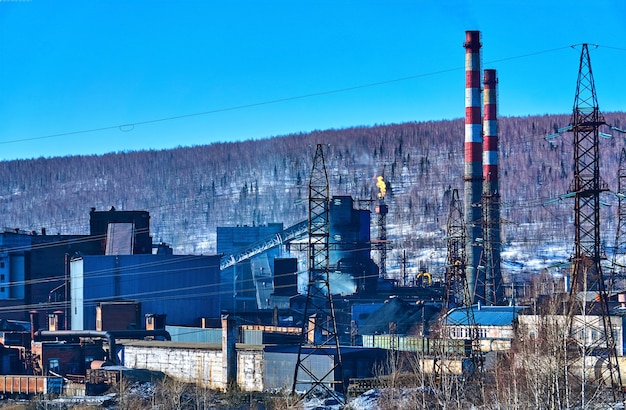This detailed image depicts an industrial complex, possibly a factory or power plant, characterized by a series of rectangular structures of varying heights and widths. The buildings are a mix of elongated single-story stone buildings and taller multi-story metal-sided constructions. Dominating the scene are two tall, conical smokestacks with alternating red and white stripes. A distinct feature is a rusted utility tower with power lines attached, and one of the steel beams has flames emerging from its top. In the foreground, a train track with a single boxcar on the left side runs parallel to the buildings, while brown grass and weeds add a touch of nature to the industrial setting. Further details include a white brick bridge or wall and several smaller buildings that people can enter. The background reveals a forested hillside and bare trees, suggesting a winter setting, with some snow visible on the ground. The sky overhead is a clear blue, indicating that the image was taken during the daytime. The image might either be a photograph or a photorealistic painting, given its detailed and realistic representation.